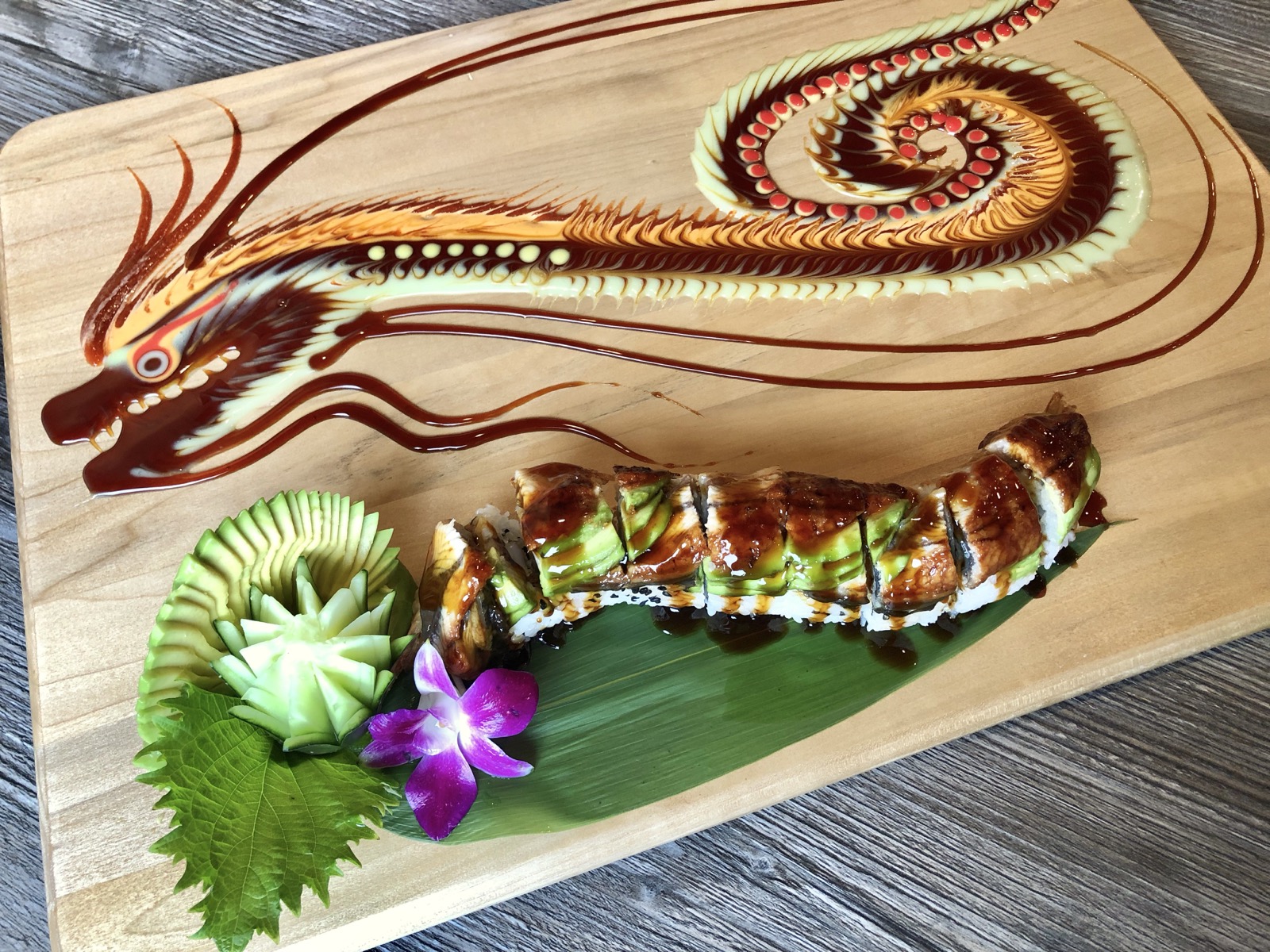This image showcases an intricate and high-end sushi presentation on a light brown wooden cutting board, set against a weathered gray wood background. The top two-thirds of the cutting board are dominated by an elaborate Asian dragon design rendered in various sauces. The dragon, featuring detailed scales, spikes along its back, and a distinguishable red eye, has been meticulously crafted using a combination of dark soy sauce, lighter mayonnaise, and possibly white mustard. The dragon's tail is adorned with small red food decorations, adding an extra layer of detail to the design.

Below the dragon, on a flat, dark green banana leaf, lies a beautifully arranged dragon roll sushi. The sushi roll is adorned with alternating slices of cucumber and fish atop a bed of rice sprinkled with black sesame seeds. The roll is artistically laid out to resemble a caterpillar, complete with a brown teriyaki-type sauce drizzled over it. To the left of the sushi roll, a cucumber spiral and a small purple flower add color and elegance to the composition, further showcasing the remarkable skill and attention to detail invested in this culinary masterpiece.